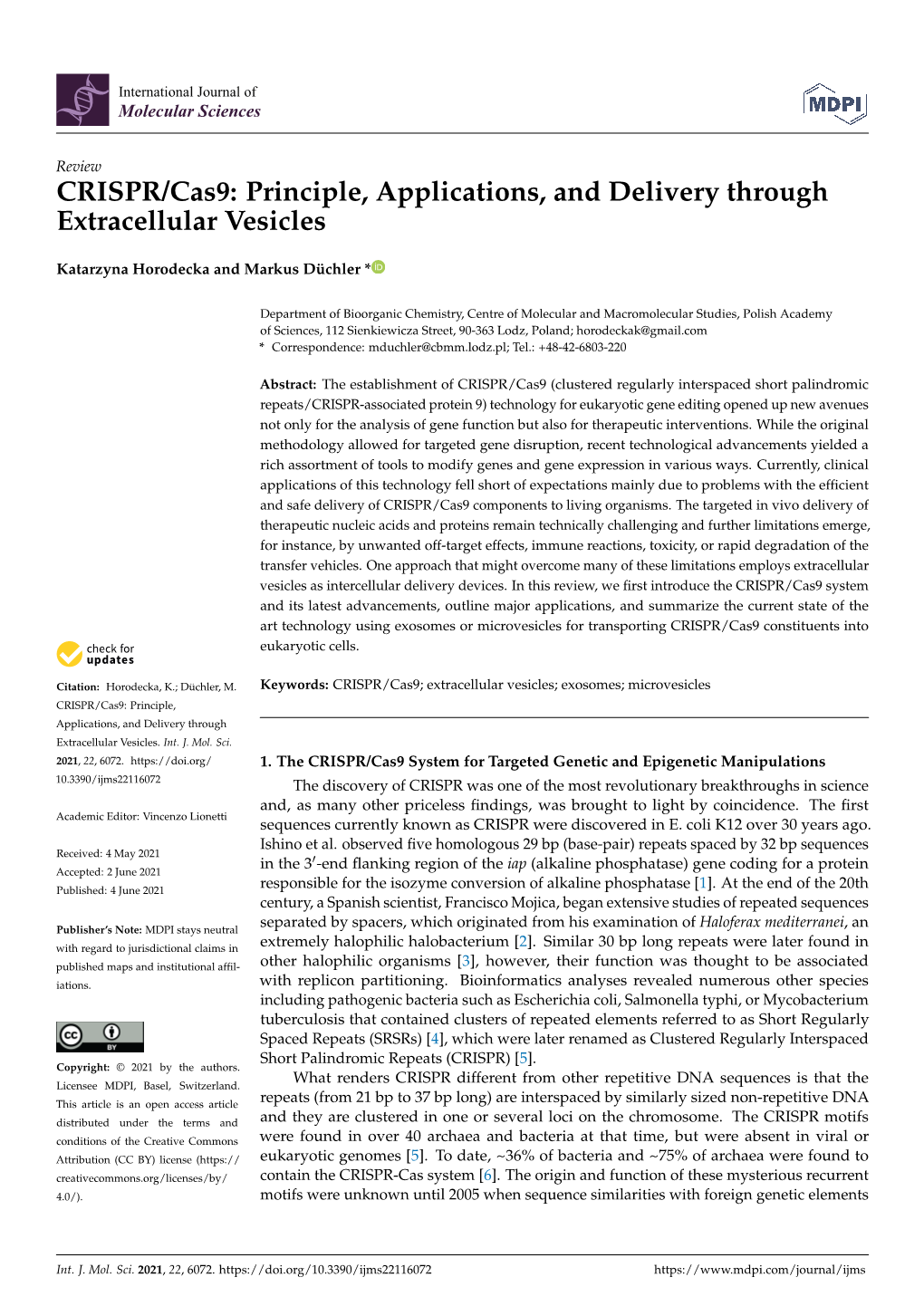The image features a white background with several distinct elements. In the upper left corner, there is a blue square containing a stylized blue DNA strand. Positioned to the right of this square, the title "Internal Journal of Molecular Sciences" appears in black text. Further to the right, there is a logo inscribed with "MDPI."

A horizontal black line divides the upper and lower sections of the image. Beneath this line, the title "Review: CRISPR/Cas9 Principles, Applications, and Delivery for Extracellular Vehicles" is prominently displayed. The authors, Cataract Horodeca and Marcus Duculler, are listed below the title.

The lower section is filled with extensive black text detailing the scientific principles and applications of CRISPR/Cas9, presented in a dense and technical manner. At the bottom of the image, two websites are noted, likely sources of additional information or references.